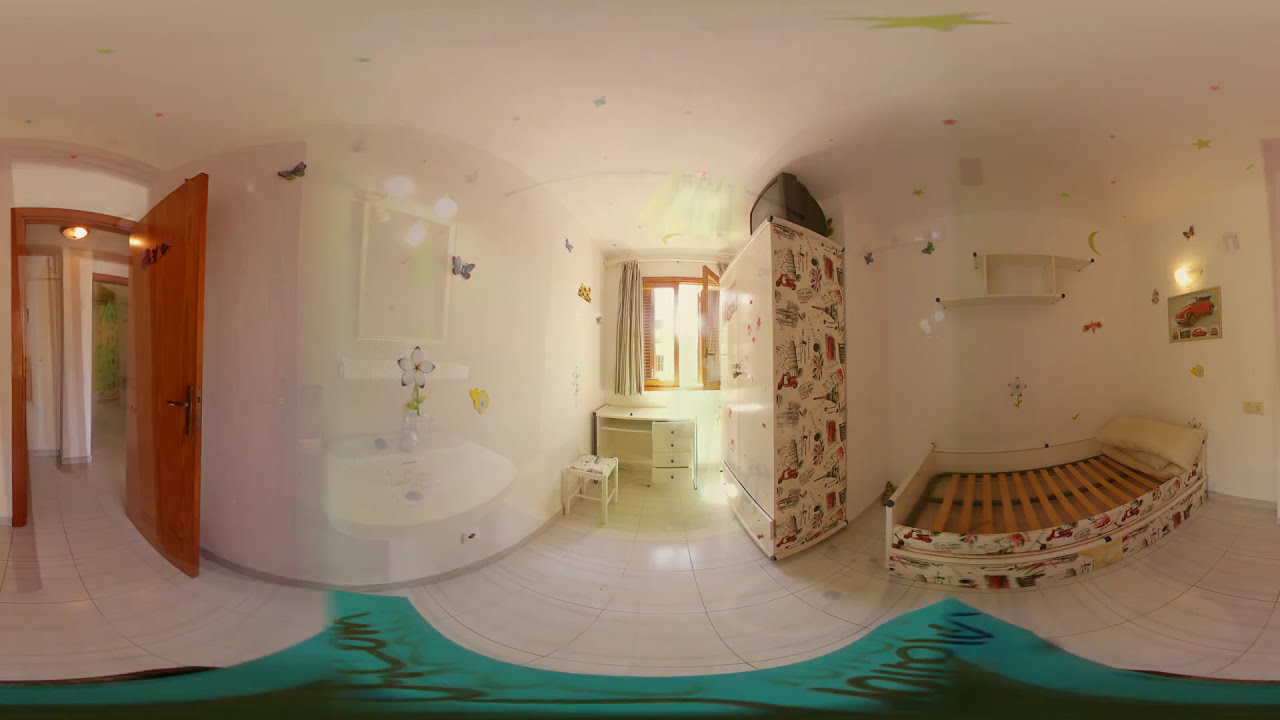The image depicts a room in an apartment or house, captured through a curved wide-angle perspective. On the right side, there is a bed frame without a mattress, showcasing wooden slats and an off-white frame adorned with unique graphic designs. A stray pillow is still on the bed frame. The white walls feature decals of butterflies and flowers, along with a photograph of a car. In the center, a cream-colored desk paired with a stool sits beneath an open, light-filled window with draperies. Above the desk, two globe light bulbs are fixed on a vanity area, possibly containing a sink. To the far left, there is a wooden door leading to other rooms. The floor is covered in white ceramic tiles.